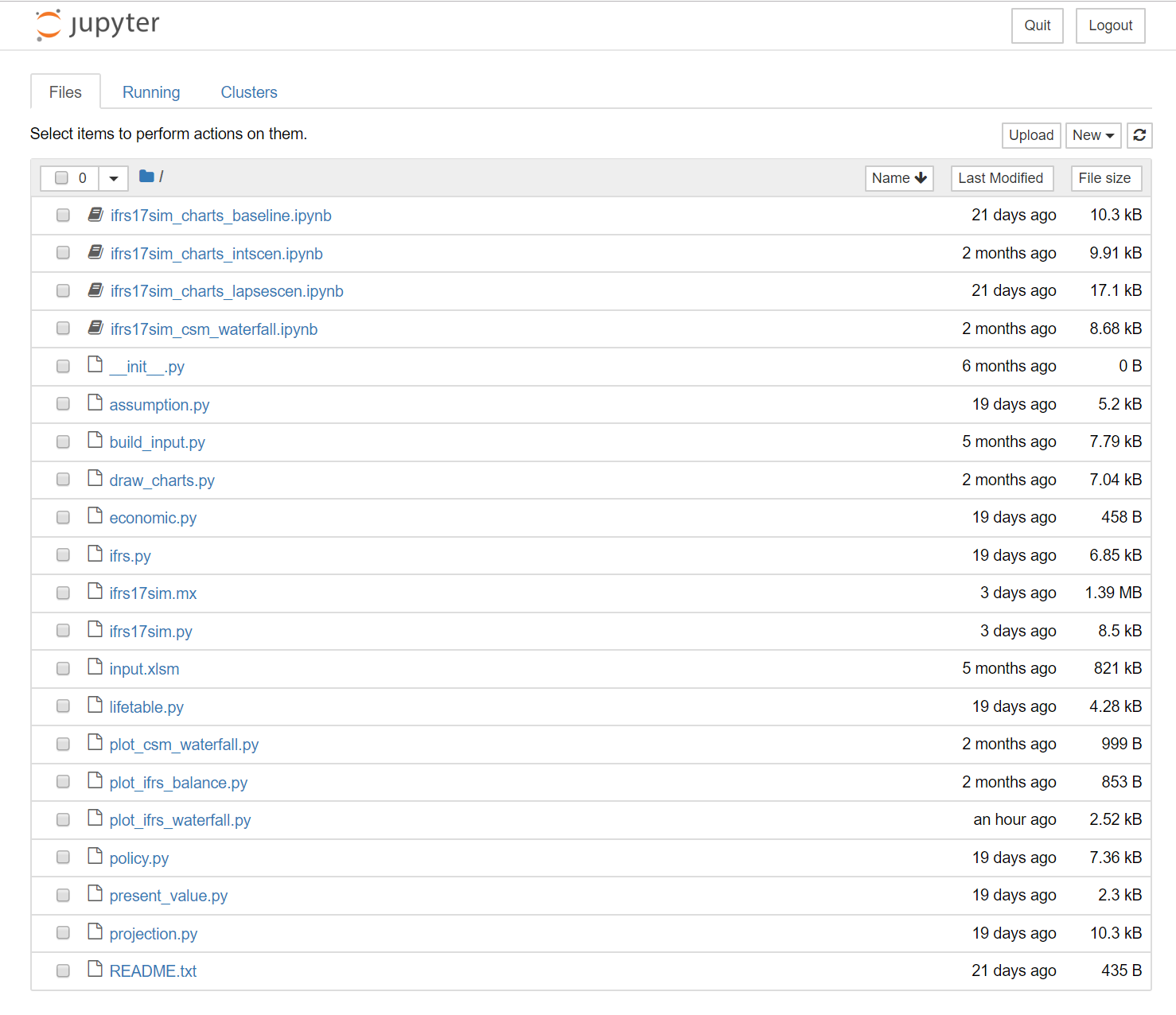**Detailed Description of the Jupyter Notebook File List Interface**

The image depicts the interface of a Jupyter Notebook file management page. On the left-hand side, the interface features the Jupyter logo, which consists of an incomplete circle reminiscent of brackets with three blue dots arranged with two at the top and one at the bottom, next to the text "JUPYTER". 

On the right-hand side, there are two buttons labeled "Quit" and "Log Out," positioned beneath each other. Below these buttons, there are three tabs, identified by the words: "Files," "Running," and "Clusters." The "Files" tab is currently active.

Directly under the tabs is a small instruction text: "Select items to perform actions on them." Adjacent to this text, on the right side, there are three action buttons: "Upload," "New" with a dropdown arrow, and the refresh icon.

Beneath these buttons, a gray header banner outlines the file list with columns titled "0" (featuring a dropdown box and a blue folder icon), "Name" with a sorting arrow, "Last Modified," and "File Size."

The files listed below this header are ordered with details as follows:

1. **IFRS17_SIM_charts_baseline.ipynb**
   - Last Modified: 21 days ago
   - File Size: 10.3 KB

2. **IFRS17_SIM_charts_INTSCEN.ipynb**
   - Last Modified: 2 months ago
   - File Size: 9.9 KB

3. **IFRS17_SIM_charts_LAPSESCEN.ipynb**
   - Last Modified: 21 days ago
   - File Size: 17.1 KB

4. **IFRS17_SIM_SIM.waterfall.ipynb**
   - Last Modified: 2 months ago
   - File Size: 8.68 KB

5. **__init__.py**
   - Last Modified: 6 months ago
   - File Size: 0.1 KB

6. **IFRS17_SIM_charts_waterfall.ipynb**
   - Last Modified: 2 months ago
   - File Size: 0.1 KB

7. **ASSUMPTION.py**
   - Last Modified: 19 days ago
   - File Size: 5.2 KB

8. **BUILD_INPUT.py**
   - Last Modified: 5 months ago
   - File Size: 7.79 KB

9. **DRAW_charts.py**
   - Last Modified: 19 days ago
   - File Size: 7.04 KB

10. **ECONOMIC.py**
    - Last Modified: 19 days ago
    - File Size: 4.58 bytes

11. **IFRS.py**
    - Last Modified: 19 days ago
    - File Size: 6.85 KB

12. **IFRS17_SIM.mx**
    - Last Modified: 3 days ago
    - File Size: 1.39 MB

13. **IFRS17_SIM.py**
    - Last Modified: 3 days ago
    - File Size: 8.5 KB

14. **INPUT.xism**
    - Last Modified: 5 months ago
    - File Size: 821 KB

15. **LIFETABLE.py**
    - Last Modified: 19 days ago
    - File Size: 4.28 KB

16. **PLOT_CSM_WATERFALL.py**
    - Last Modified: 2 months ago
    - File Size: 9.99 bytes

17. **PLOT_IFRS_BALANCE.py**
    - Last Modified: 2 months ago
    - File Size: 8.53 bytes

18. **PLOT_IFRS_WATERFALL.py**
    - Last Modified: 1 hour ago
    - File Size: 2.52 KB

19. **POLICY.py**
    - Last Modified: 19 days ago
    - File Size: 7.36 KB

20. **PRESENT_VALUE.py**
    - Last Modified: 19 days ago
    - File Size: 2.3 KB

21. **PROJECTION.py**
    - Last Modified: 19 days ago
    - File Size: 10.3 KB

22. **README.txt**
    - Last Modified: 21 days ago
    - File Size: 435 bytes

This descriptive list provides a clear and detailed overview of the layout and the files available on the Jupyter Notebook interface.